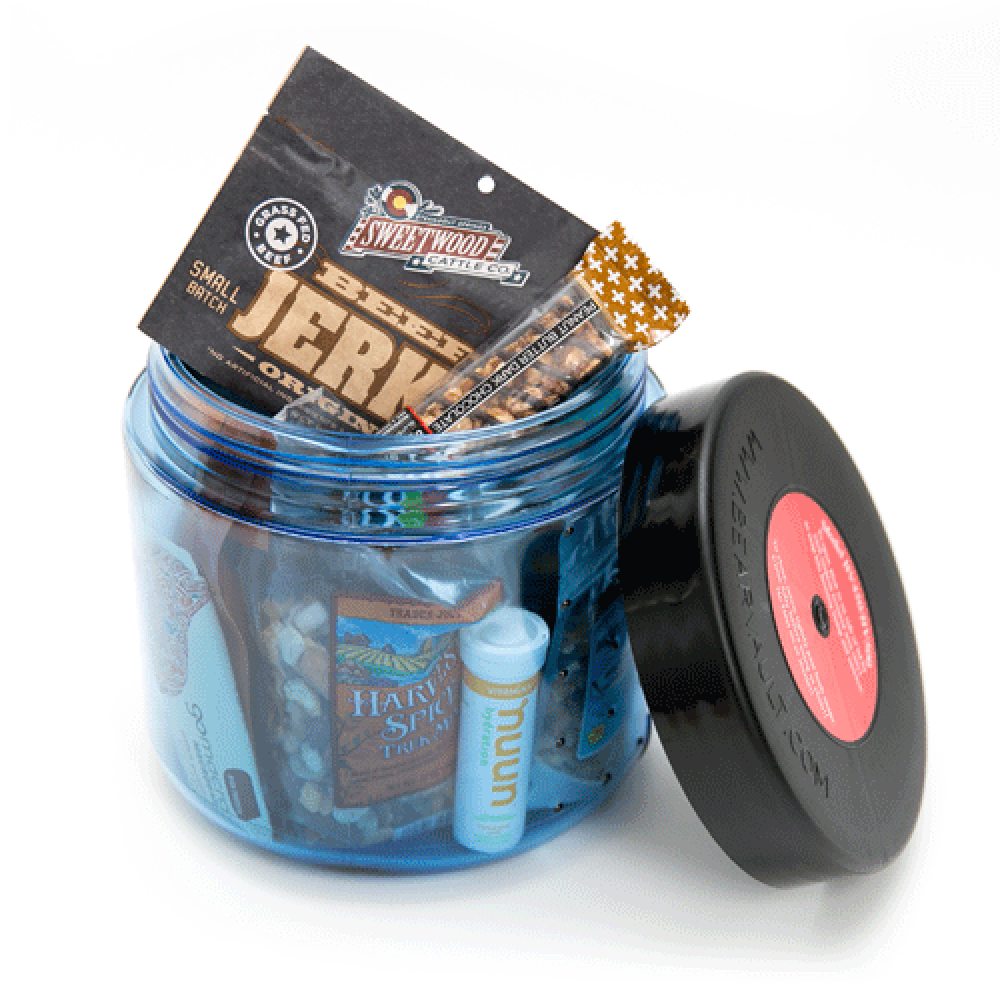The image showcases a collection of healthy snacks inside a container designed for protein-rich nourishment. Featured prominently is a package of Streetwood Cattle Company beef jerky, noted for its small-batch, grass-fed beef. Alongside it, there's a KIND bar, flavored with peanut butter and dark chocolate. A bag of Harvest Spice Trail Mix, sourced from Trader Joe's, adds a seasonal touch with its blend of spices and nuts. Also included is a packet of Nuun, presumably a sports beverage or energy powder, though its exact purpose remains unclear. Completing the assortment is a GoMacro bar, commonly known for its wholesome, nutrient-packed ingredients. Overall, this container seems to be curated for those seeking a variety of protein-rich, health-conscious snacks.